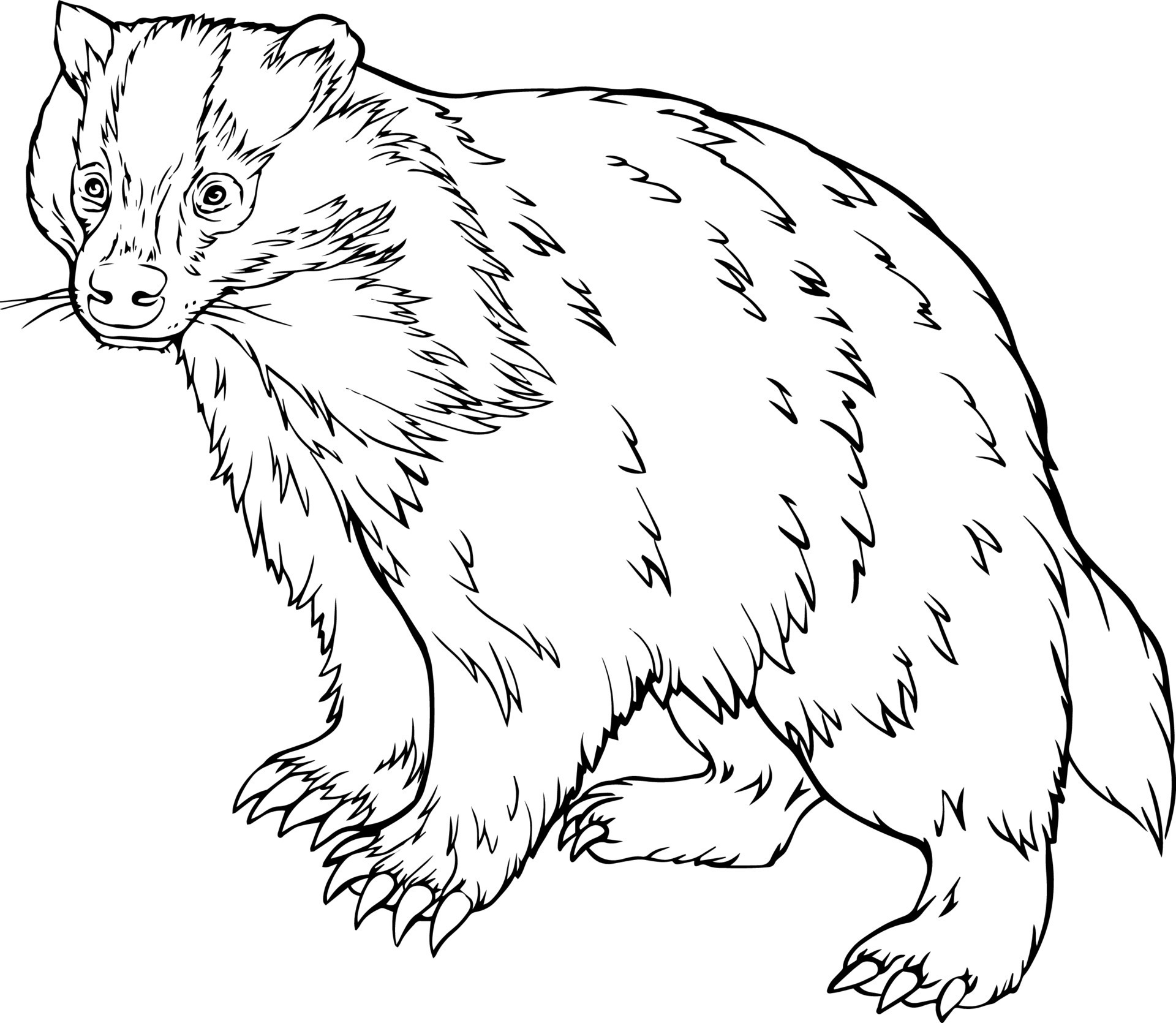The image is a black and white hand-drawn sketch of a skunk, meticulously outlined in black with numerous V-shaped lines that depict a detailed fur pattern. The skunk is oriented to the left side of the image, featuring a nose that mimics the shape of a capital letter "I" and two small eyes. Its mouth has whiskers, accentuating its facial features. Each of its front legs has four sharp, needle-like claws, while the back legs have three similar claws. The skunk's body is predominantly covered in shaggy fur, extending around the neck and head. A short, bushy tail is positioned to the right side of the image. The drawing, rendered entirely in black ink, lacks color, which contributes to its somewhat ambiguous appearance, leading to initial misidentifications as other animals such as a groundhog, gopher, or wolverine.